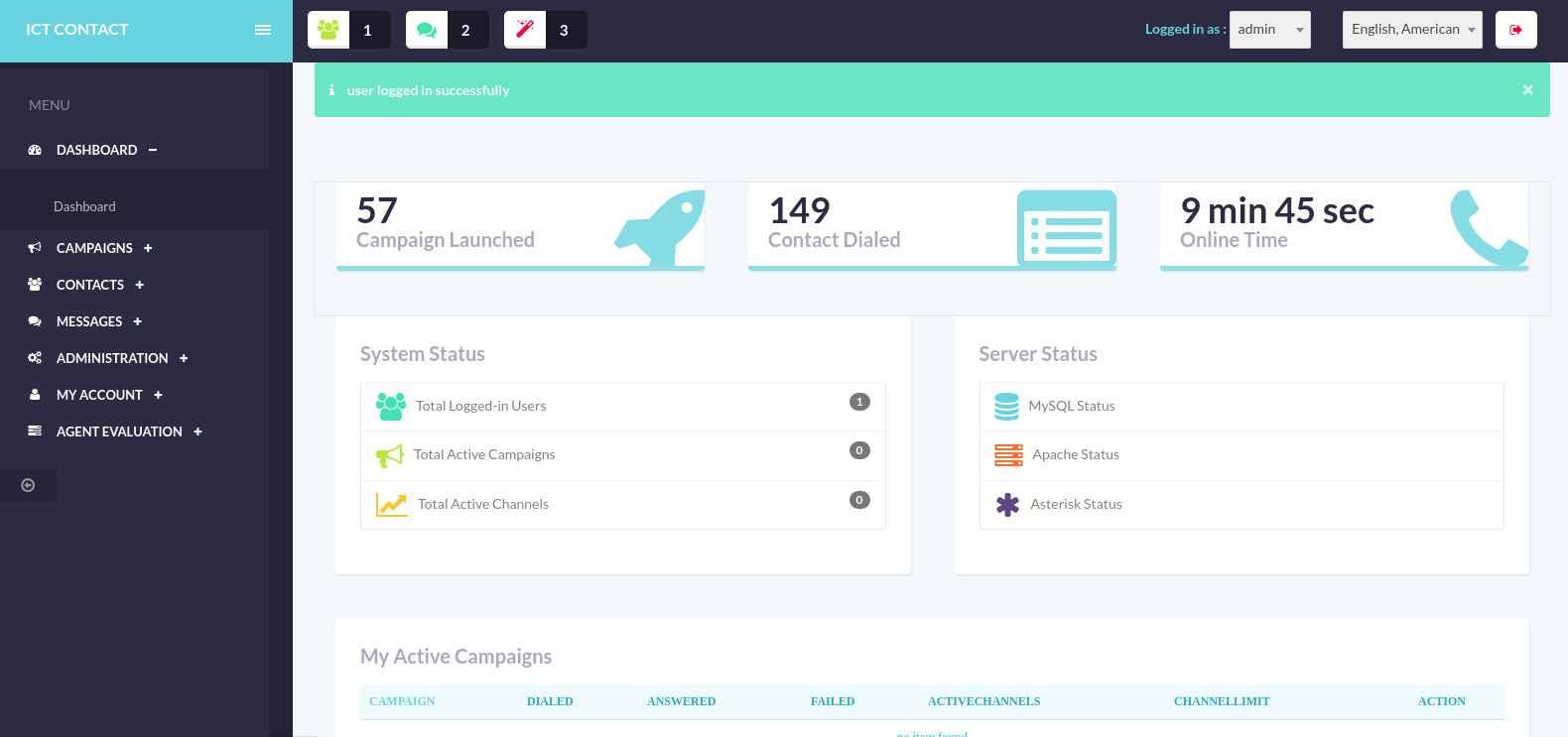This screenshot captures the interface of a website's dashboard. At the top, we see the section labeled "Key," with the term "ICT Contact" prominently displayed in teal. Adjacent to it, in black, are menu options including "Menu," "Dashboard," "Campaigns," "Contacts," "Messages," "Administration," "My Account," and "Agent Evaluation," each accompanied by an icon on the left.

On the right side of the screen, a green notification box states "User logged in successfully." Below this notification, user statistics are displayed: "57 campaigns launched," "149 contacts dialed," and "9 minutes and 45 seconds online time."

Towards the bottom of the screen, under the section labeled "System Status," we see details such as "Total logged in users: 1," "Total active campaigns: 0," and "Total active channels: 0." To the right, a rectangular box titled "Server Status" provides further technical information, including "MySQL status," "Apache status," and "Asterisk status."